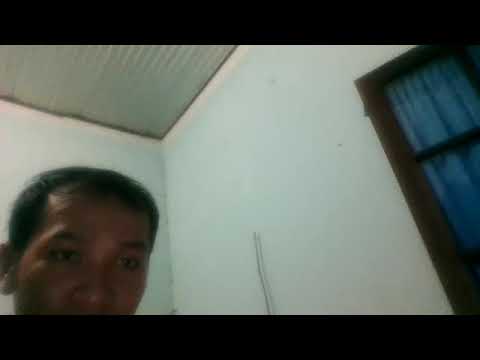This image, framed by thick black bars at the top and bottom, appears to be a still shot from a video. It features a man with dark brown, shiny skin and short black hair, looking slightly to the right while his head faces forward. His facial features include black eyebrows, visible ears, and a broad nose. The man is captured in what seems to be a corner of a room. The intersecting walls are a light turquoise seafoam green, while the ceiling, which has a striated or wavy texture and a brown border, appears slightly darker. On the right side of the image, there is a portion of a black door with a grid pattern, adorned with a bright blue curtain. The captured environment hints at a domestic interior, potentially a home.